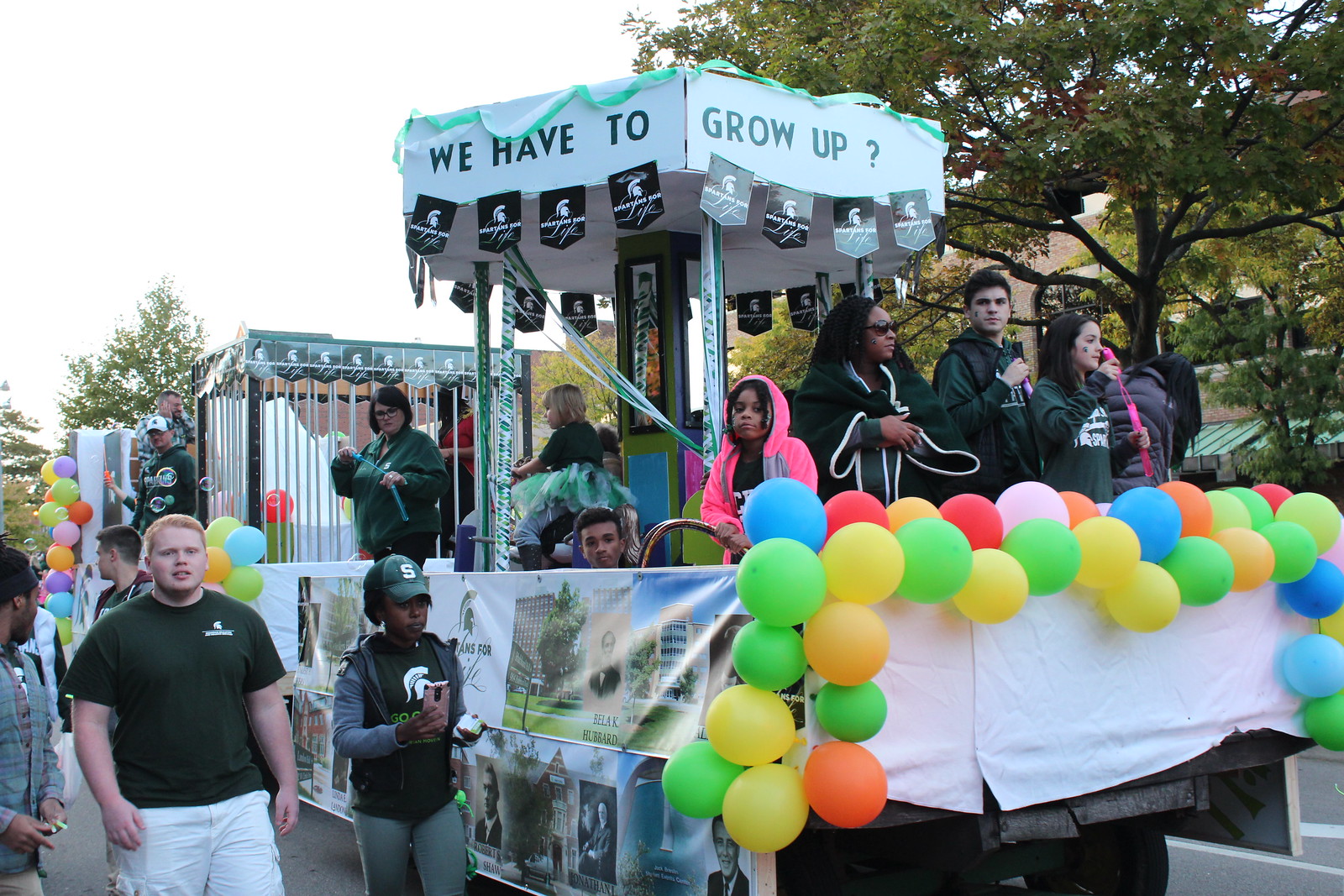The image captures a lively parade scene featuring a float adorned with an array of multicolored balloons at its front. The participants and onlookers, a diverse mix of ages and ethnicities, are dressed in green shirts and black robes, while one standout youngster dons a pink hoodie. People are seen walking alongside the float, which has a striking display reading "We have to grow up?" at the top. Central to the float is a charming gazebo where some individuals are seated, and the rear features a cage-like structure reminiscent of an enclosure for animals, integrated into the float's design. The float and participants' outfits are embellished with various logos and emblems, though too small to decipher. Bright balloons in shades of red, yellow, green, pink, and orange add to the festive atmosphere, while additional Spartan helmet decorations dangle from the float. In the background, trees and other parade floats are partially visible, hinting at the grander scale of the event. This scene suggests a parade organized by possibly a school community, meant to convey a message of growth and development.